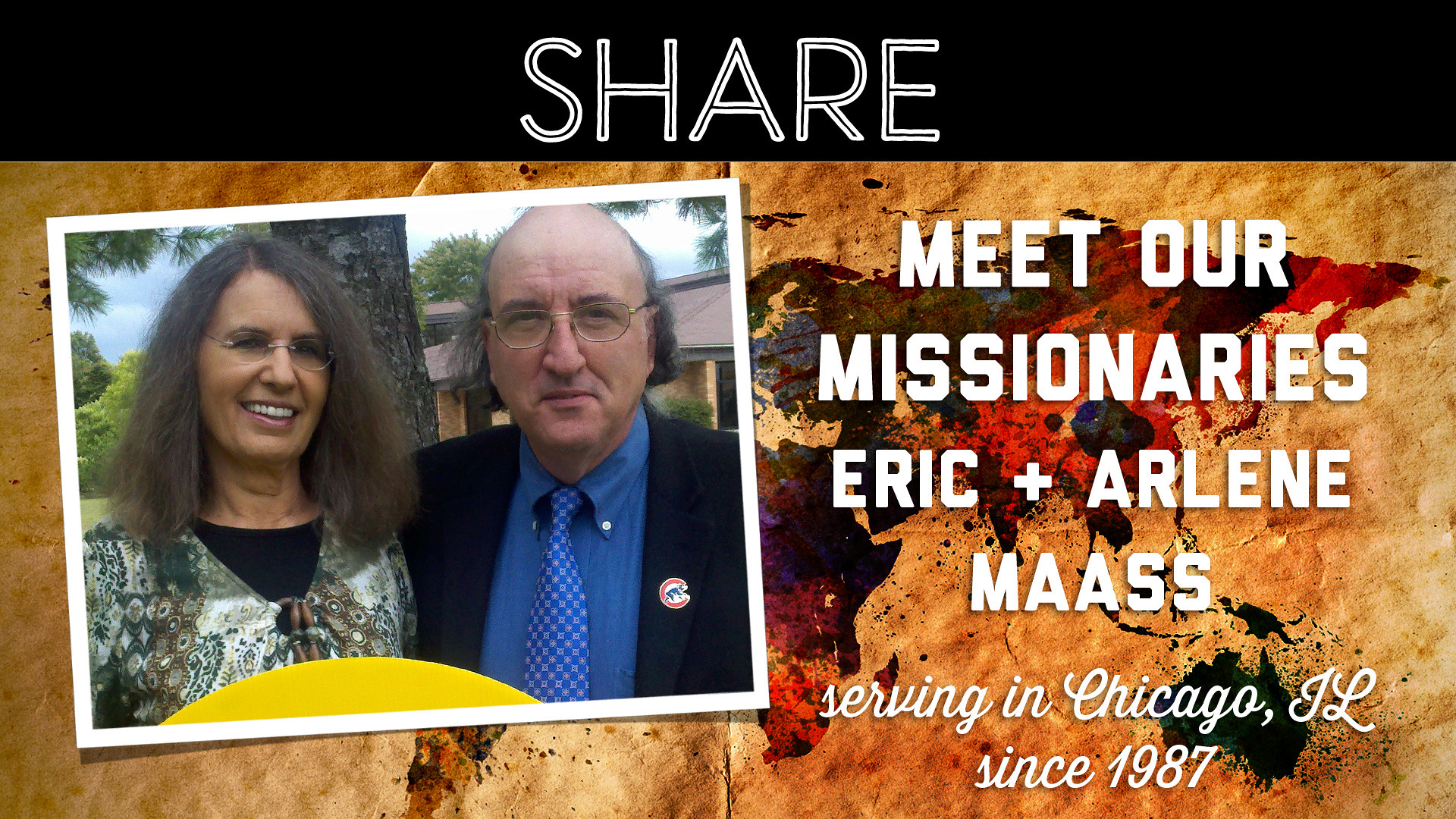The image features a rectangular banner advertisement with a black bar across the top, displaying the word "SHARE" in bold white capital letters. Below this, the background resembles old parchment with a painted world map depicting Australia, Asia, and Africa in watercolor hues of reddish-yellow and purplish-green. On the left side of the image, a photograph with a white border showcases an elderly couple smiling at the camera. The man, balding with glasses, is dressed in a black blazer with a blue shirt and tie, and a badge of a sea emblem on his blazer. The woman beside him has gray-brown hair, brown skin, and wears glasses along with a green dress layered over a black t-shirt. Behind them, a tree and houses are visible. To the right of the photograph, the text in white capital letters introduces the couple: "MEET OUR MISSIONARIES, ERIC AND ARLENE MASS," with a caption below in italics that reads, "Serving in Chicago, IL since 1987."